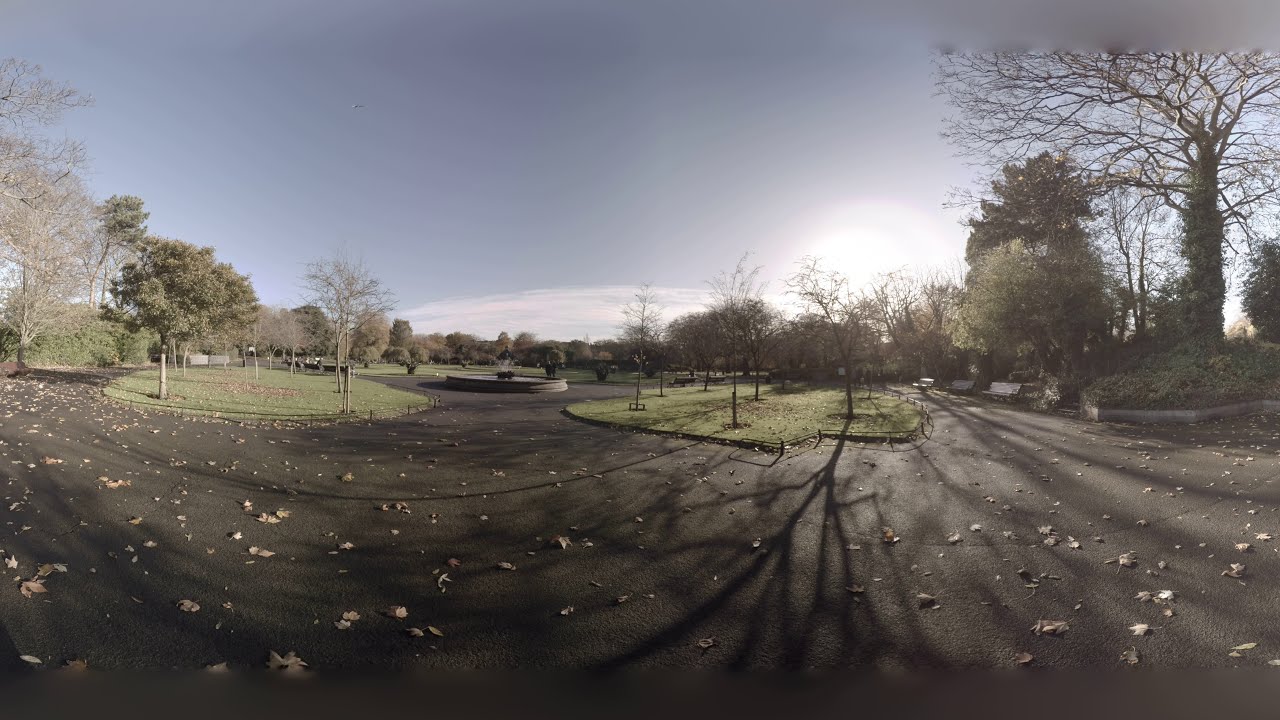The image depicts an outdoor scene set in the middle of the day during autumn. The foreground features a gray asphalt road, scattered with numerous leaves hinting at an autumn setting. Central to the image are various grassy islands with trees, many of which are bare, highlighting the season. The smaller trees are interspersed within these grassy patches, while a notable barren tall tree stands on the far right, surrounded by some evergreen pine trees.

On the left side of the image, there's a round fountain with water spouting from its center. Adjacent to this, there is an area of pavement and more grassy islands. Benches can be seen along the edges of the roadway, which enters from the bottom right of the image and arcs upwards. The sky is mostly clear with a few whitish clouds, creating an arc pattern near the center, letting through rays of sunlight that illuminate the scene. In the distant background, patches of green grass and bare trees are visible. There may be faint outlines of a fence and additional benches, adding depth to the scenery. Overall, the scene is a tranquil snapshot of a partly cloudy day in autumn within what appears to be a parking lot or a park setting.